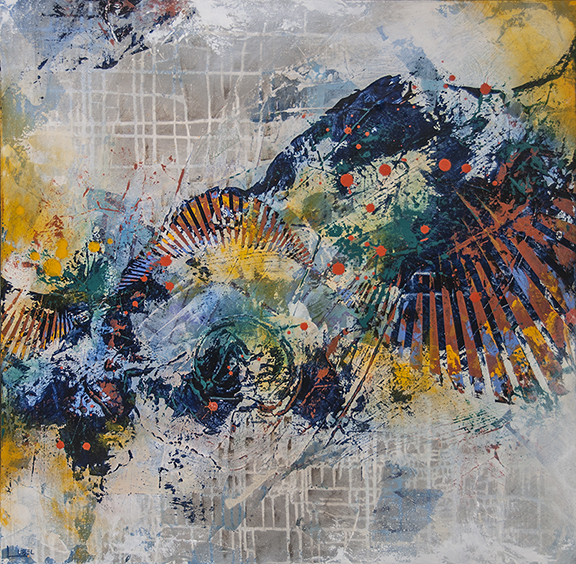This abstract art piece features a dynamic composition with multiple layers of paint, creating a striking impression of movement and depth. The background layer presents a light gray canvas intricately marked with white lines, resembling a grid or a drip pattern. Overlapping the backdrop, there are vibrant swathes of orange, green, blue, yellow, and red, arranged in forms that evoke both wing-like shapes and the imagery of a wooden bridge seen from an unusual angle. These colored elements generate a feeling of organic motion, further intensified by the directional slant from left to right. Some viewers might interpret the composition as an eagle with its wings spread wide, descending over a snow-capped mountain range, while others might see an array of tree branches or limbs adorned with white splotches, akin to blooming flowers. The topmost layer of the painting features scattered drops of red paint, adding an element of raw dynamism against the myriad of vivid colors and pale hues beneath. This layered complexity and interplay of colors render the piece a captivating blend of abstraction, suggesting multiple interpretations and emphasizing its vibrant, ever-changing nature.